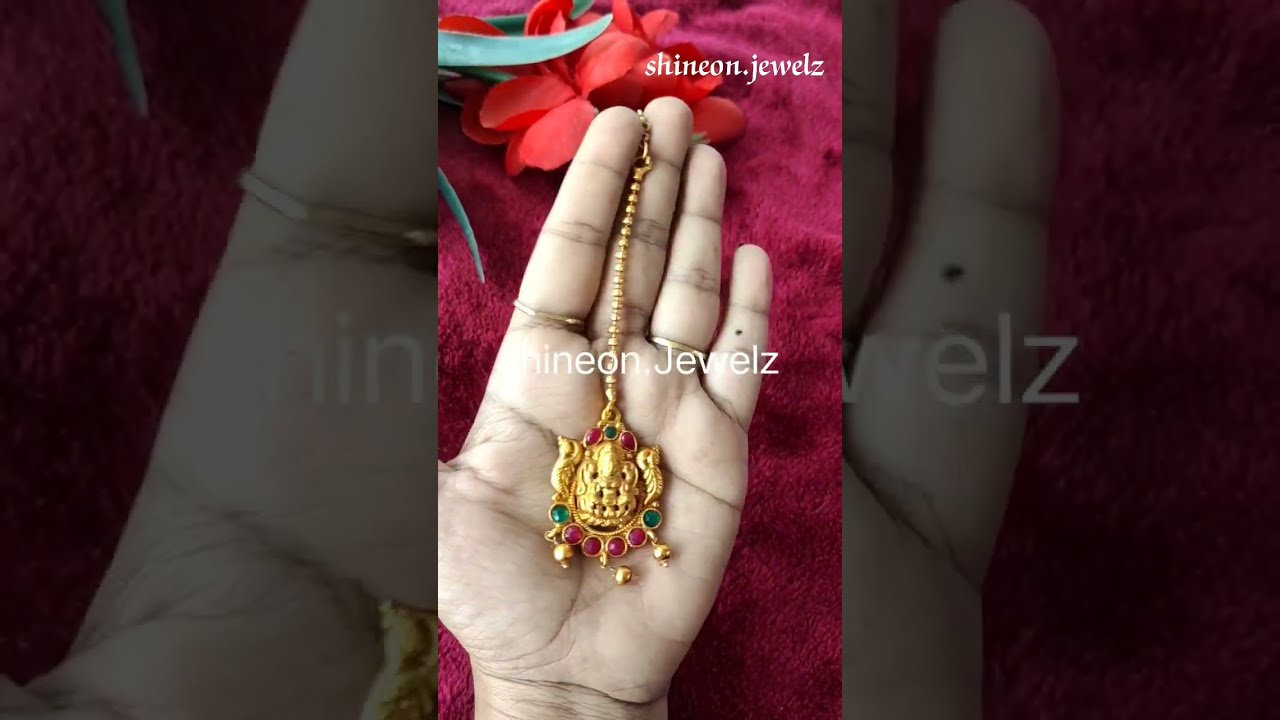In the image, an extended human hand, centered against a maroon, furry surface, holds an ornate piece of gold-colored jewelry, known as a plantum. The open palm showcases the plantum, which features intricate designs with small beads on top and an array of green and pink beads along its circular base, with golden beads hanging beneath. The detailed backdrop includes a striking red flower at the top and some greenery peeking through, reinforcing the indoor setting of the photograph. Across the top of the image, the text "Chenine Jewels" is prominently displayed, reinforcing the impression that this image serves as an advertisement, possibly captured from a social media platform.